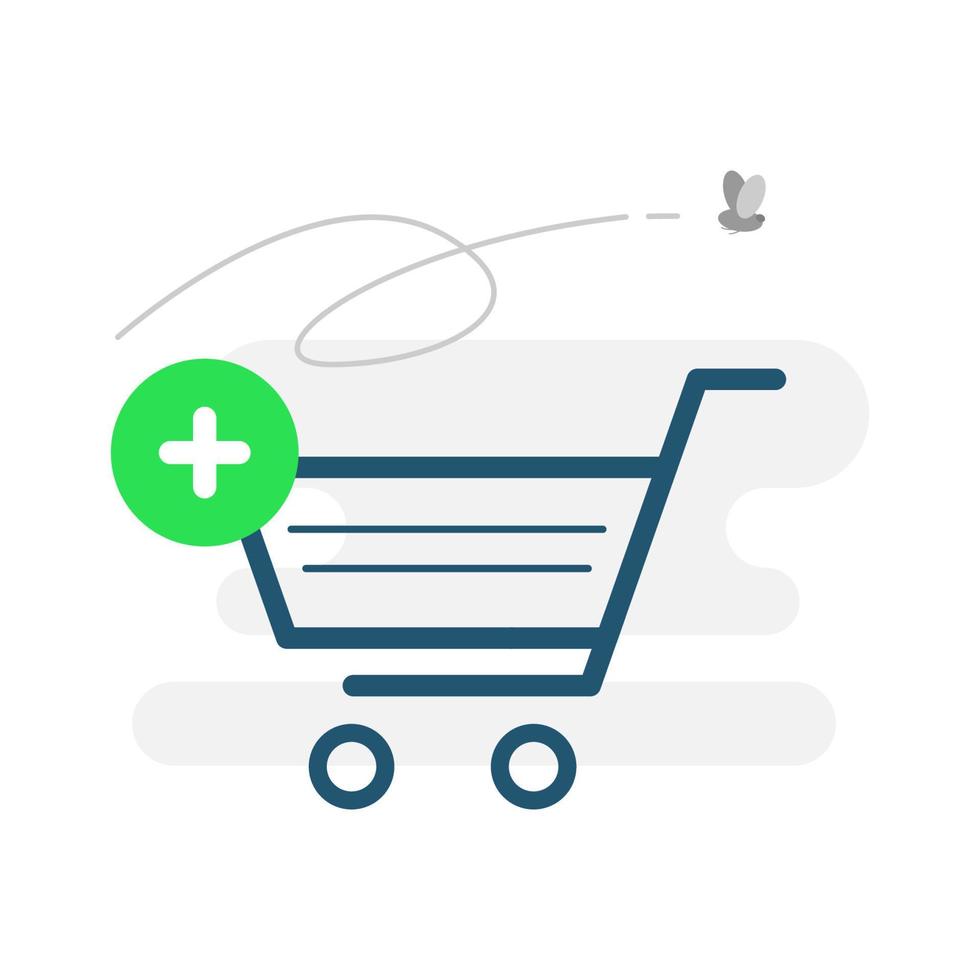The image displays a stylized logo that resembles a blue shopping cart, similar to those found in online shopping applications like Instacart. The cart, depicted in blue, features a large green circle with a white plus sign on its front, perhaps indicating the option to add items to the cart. Above the cart, a bee or fly is illustrated in gray, with a swirling line tracing its path back to the cart, adding a sense of motion. Behind and around the cart are two light blue abstract shapes, one elongated and the other otter-shaped, enhancing the overall design. This logo appears to symbolize a dynamic and user-friendly shopping experience.